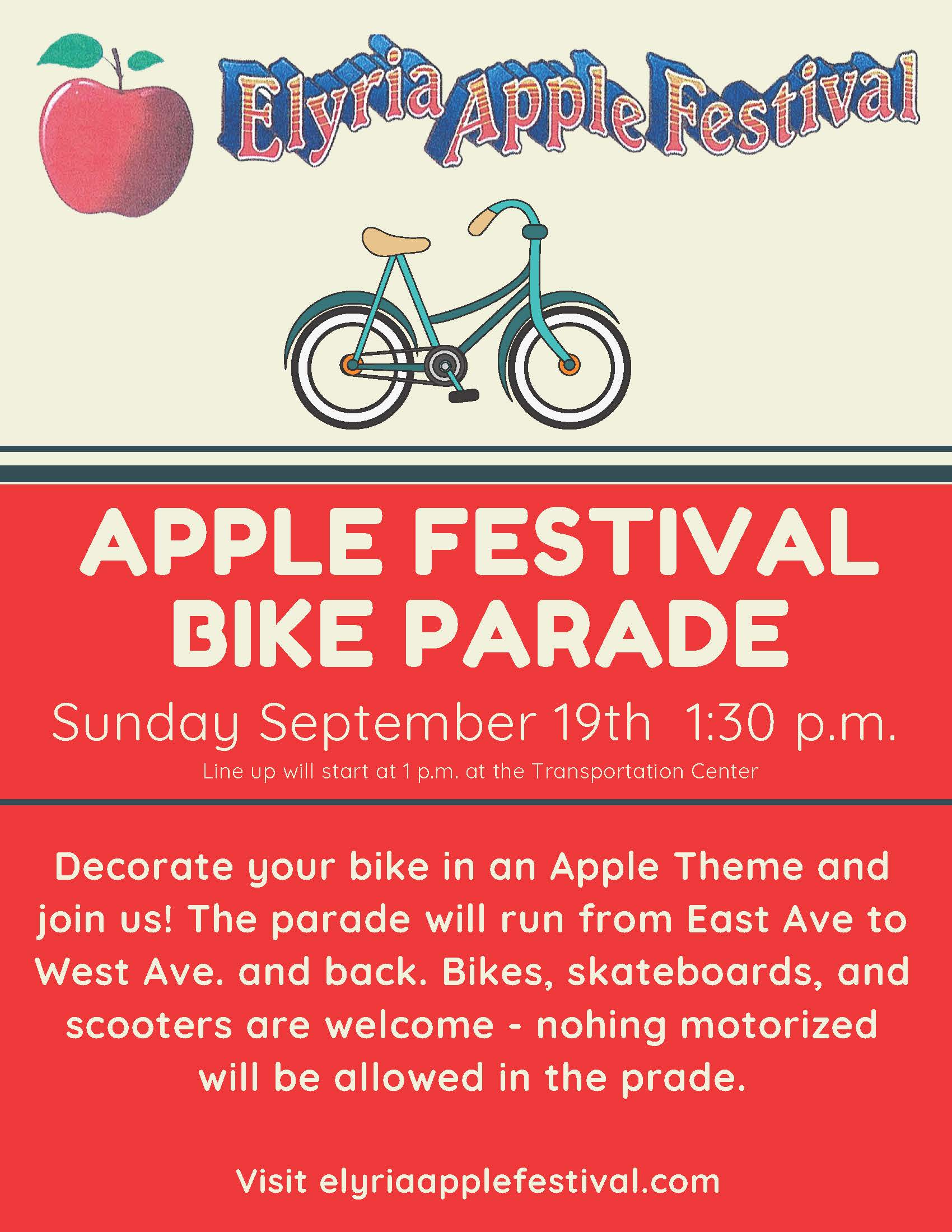This vibrant poster is an advertisement for the Aliria Apple Festival, prominently titled in bold red lettering at the very top. On the left side, there's a detailed illustration of a red apple with a stem and green leaves. Below the apple, an aqua-colored and yellow bicycle with black and white wheels is depicted. Beneath the bicycle, a red block with white letters announces the "Apple Festival Bike Parade, Sunday, September 19 at 1:30 PM." It also specifies that the lineup will start at 1 PM at the Transportation Center. A black line separates this section from another red block with white text that encourages participants to "decorate your bike in an apple theme and join us." The parade route will stretch from East Avenue to West Avenue and back, welcoming bikes, skateboards, and scooters but explicitly stating that nothing motorized is allowed. Towards the bottom, the URL for more information is displayed: "visit aliriaapplefestival.com."